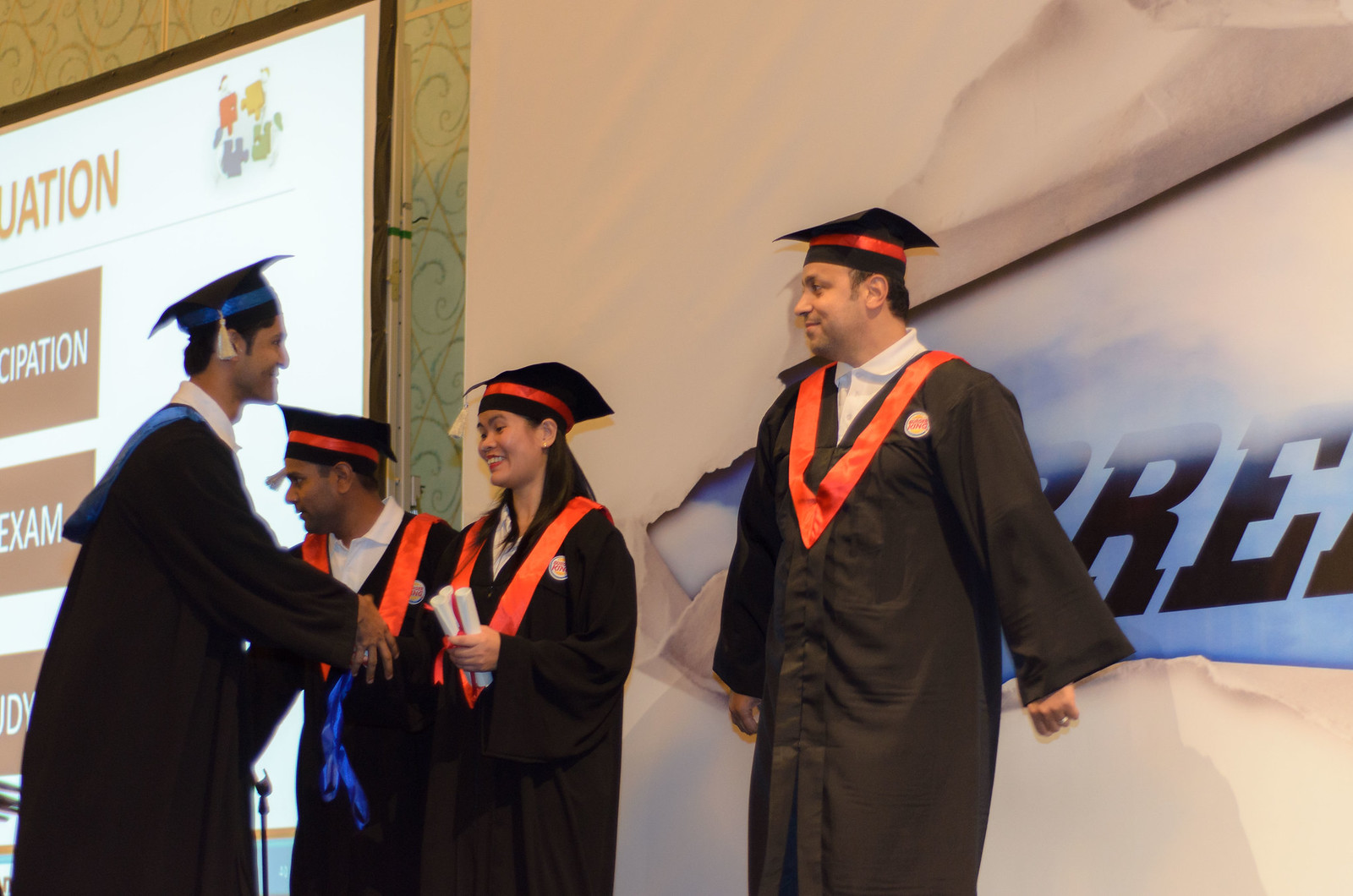In a brightly lit auditorium adorned with graduation decorations, a group of three graduates—two men flanking a woman—are captured as they step on stage to receive their diplomas. They wear traditional black gowns and caps adorned with distinctive orange tassels and sashes that form a V-shape in the front. The woman, standing center, beams happily as she shakes hands with a man donning similar graduation attire but distinguished by blue accents on his tassel, sash, and cap. Behind them, a large projection screen displays words such as "graduation," "participation," "exam," and "study," while an artistic backdrop featuring an image of paper being theatrically ripped open adds to the celebratory ambiance. The scene brims with joy and formality, capturing a significant milestone in the graduates' lives.